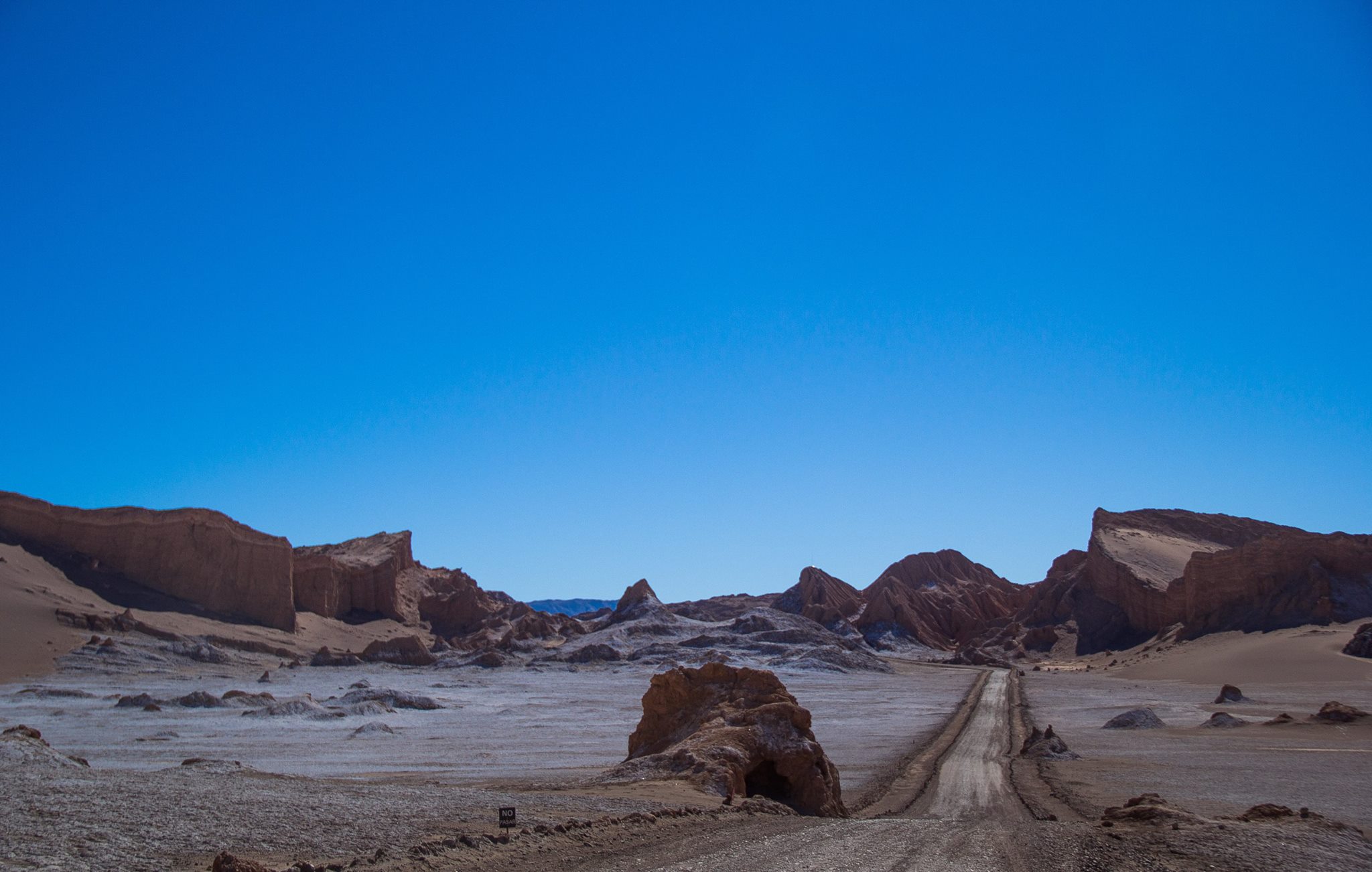The image captures an expansive outdoor setting dominated by large dirt mounds and massive rocks, giving the scene a rugged and untamed appearance. The ground is a mix of dirt and mud, with evident tracks and formations carved into the soft earth. The sky is a vibrant, bright turquoise blue, devoid of clouds, adding to the starkness of the scene. In the background, jagged dark brown cliffs rise, though they could also be described as enormous rock formations rather than true mountains. A narrow vertical pathway cuts through the sandy ground, adding depth and dimension to the landscape. The overall atmosphere is one of a bright, clear day, with an uninterrupted blue sky stretching across the horizon.